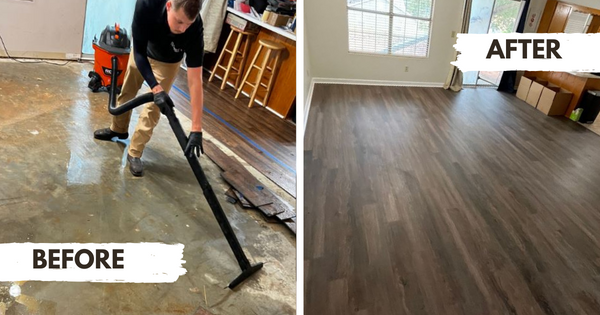This image set consists of two square color photographs illustrating a dramatic transformation labeled "before" and "after." The "before" image depicts a cluttered kitchen area undergoing repair, possibly due to water damage as evidenced by the man who is vacuuming the wet subfloor with a shop vac. The man, wearing a black uniform t-shirt, black latex gloves, and khaki pants, is focused on the task, surrounded by a disassembled setting where the engineered hardwood floor has been removed. In the background, a few bar stools face a kitchen counter covered in miscellaneous items, and an open door reveals an exterior view. The "after" photo presents a stark contrast, showcasing a pristine kitchen with shiny, dark oak laminate flooring professionally installed over the previously bare and waterlogged subfloor. The kitchen appears spotless and organized, with the bar counter tidied up and the scenery outside brightly illuminated by daylight, enforcing the impressive improvement from a damaged to a restored, aesthetically pleasing kitchen space.